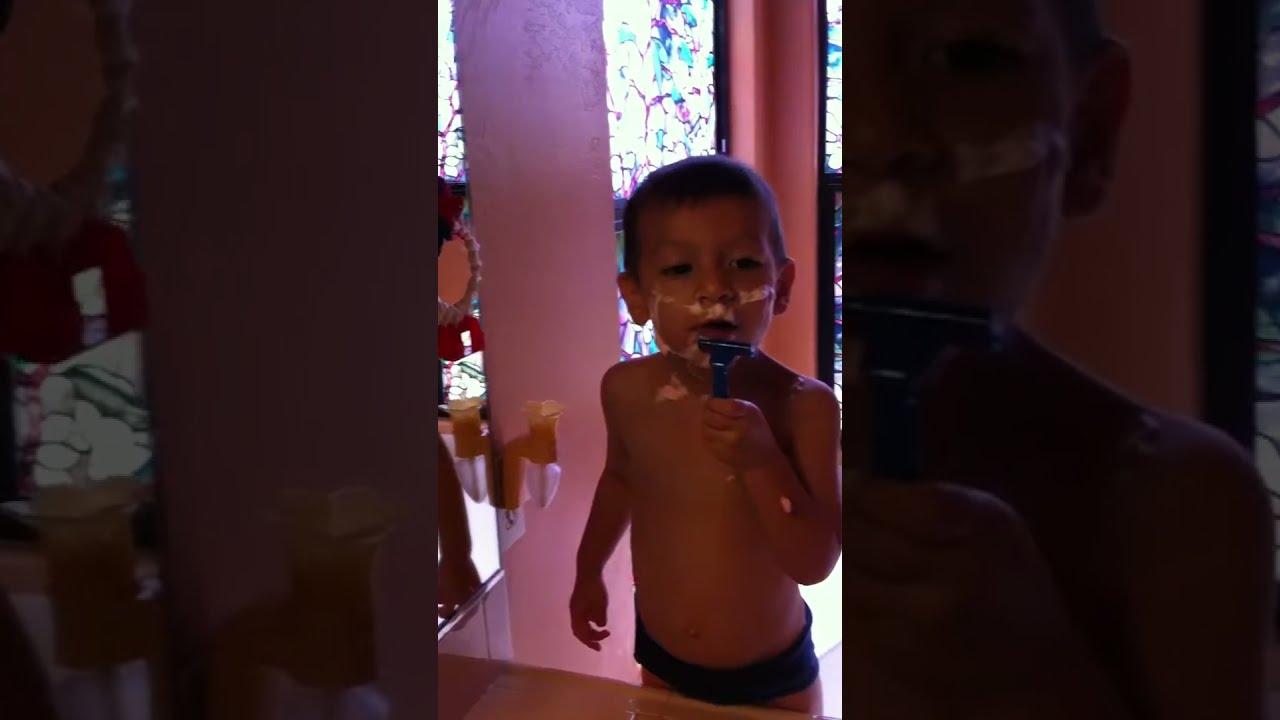In this captivating image, a little boy with brown hair and dark eyes is pretending to shave his face. His cheeks and chin, as well as a bit of his upper body and arm, are lathered with white shaving cream. Holding a blue razor in his left hand, he stands shirtless, revealing his dark blue underwear in the mirror seen to his left. The boy appears to be deeply engrossed in his playful mimicry, looking slightly to his right. 

The mirror not only reflects his intense focus but also reveals a small night lamp and another small mirror hanging within its frame. Behind him, a vibrant stained glass window, adorned with shades of purple, white, and blue, complements the eclectic decor of the room. The walls surrounding him are tinged with hues of orange, pink, and purple, adding a whimsical touch to the scene. Additionally, just beneath the mirror, there appears to be a tiled image partially visible, enhancing the intricate background details. This image beautifully captures the innocence and imaginative play of childhood.